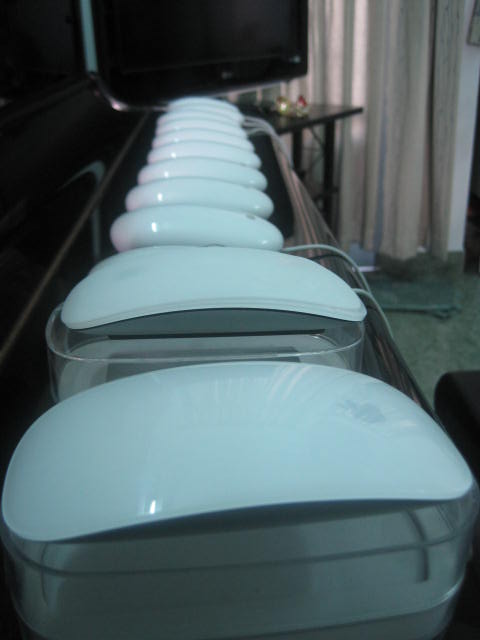The photograph captures a room featuring a dark gray carpet and a black TV that is turned off, positioned on a black stand. To the right of the TV, a light gray curtain hangs down, suggesting the presence of a window. In the foreground, there is a black counter from which a row of roughly ten to twelve glossy, white items resembling computer mice are displayed. Some of these items have cords attached, extending downward to the floor. The identities of these objects remain unclear, although their shapes and shiny surfaces stand out prominently in the image. Various unidentifiable items are also situated beside the TV.